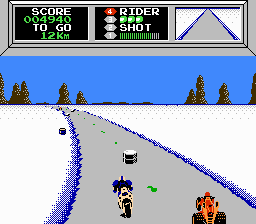The image is a screenshot from the classic video game, Mock Rider. The scene features a racetrack flanked by snow banks on both sides, with a blue sky and treeline visible at the horizon. The road curves from the bottom left corner toward the right, with two vehicles in motion: an orange, wide motorcycle on the left and a narrower, beige and black motorcycle on the right. A barrel obstacle is positioned in the middle of the road. The interface at the top of the screen displays various game statistics within a gray-bordered scoreboard. It reads "SCORE 004940" in green, followed by "TO GO 12 KM" in white, indicating the distance left to travel. Below, it shows "RIDERS LEFT 4", with three green helmets and "SHOT" highlighted. Additionally, there is a smaller inset showing an overhead view of the road and upcoming obstacles. The pixelated nature of the graphics underscores its retro, low-resolution charm.